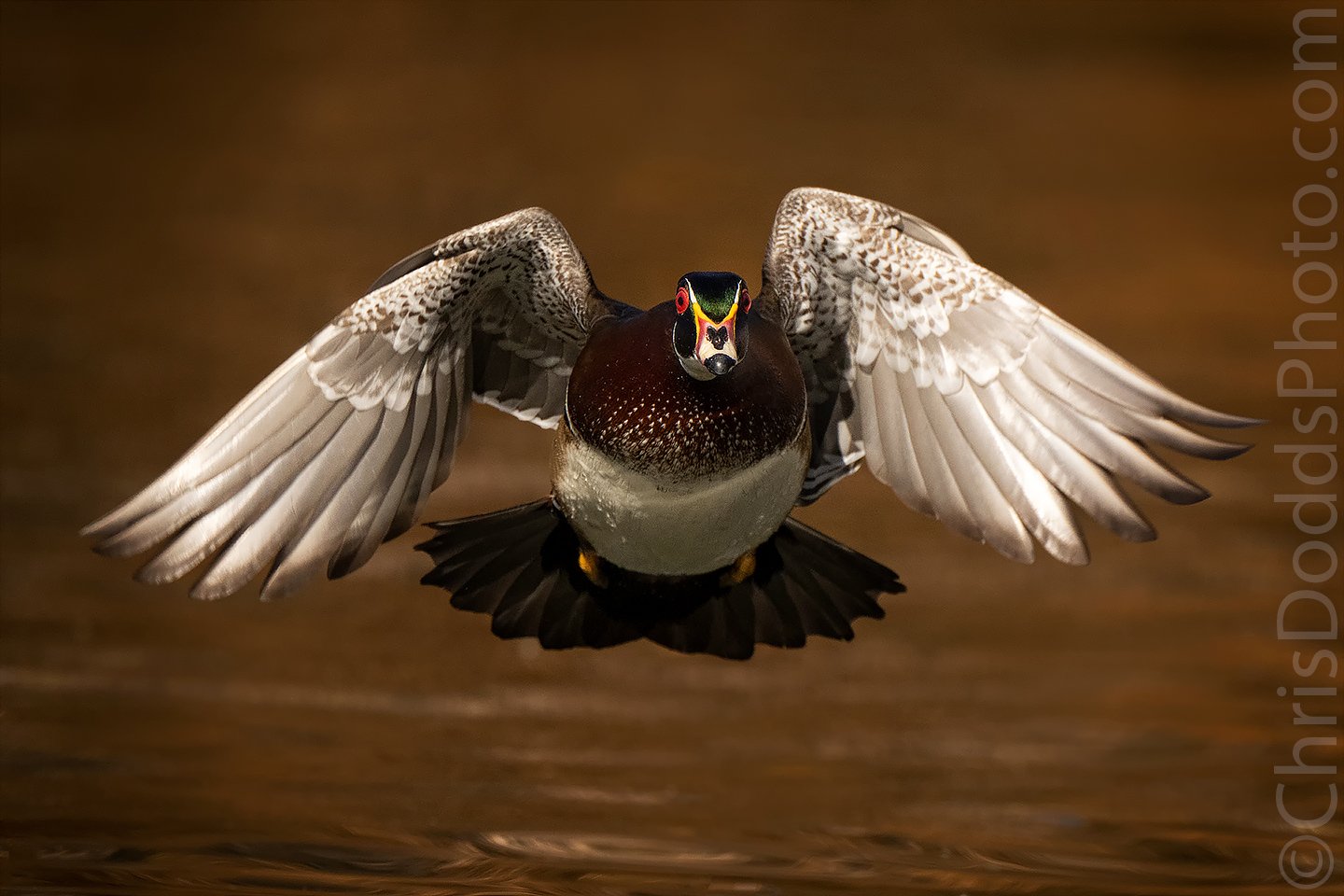The image captures a majestic bird in mid-flight, prominently featured in the center of this landscape-oriented photograph. The bird, which resembles a mallard, boasts an array of vibrant colors despite the muted brown background. Its large, outstretched wings are primarily white with light brown tips, giving them an angelic appearance. The bird displays a complex palette: its green forehead transitions to a dark head with black spots, accompanied by red eyes circled in yellow. Distinctively, the neck has a white feathered ring leading into a dark brown chest speckled with white, continuing to a fully white underbelly and a black tail. Yellow webbed feet are tucked beneath its body as it appears to be diving. The image, with minimal color aside from the bird, emphasizes its striking features. Along the right side, the watermark “ChrisDoddsPhoto.com” and the photographer's copyright are visible, crediting Chris Dodd for the photograph.